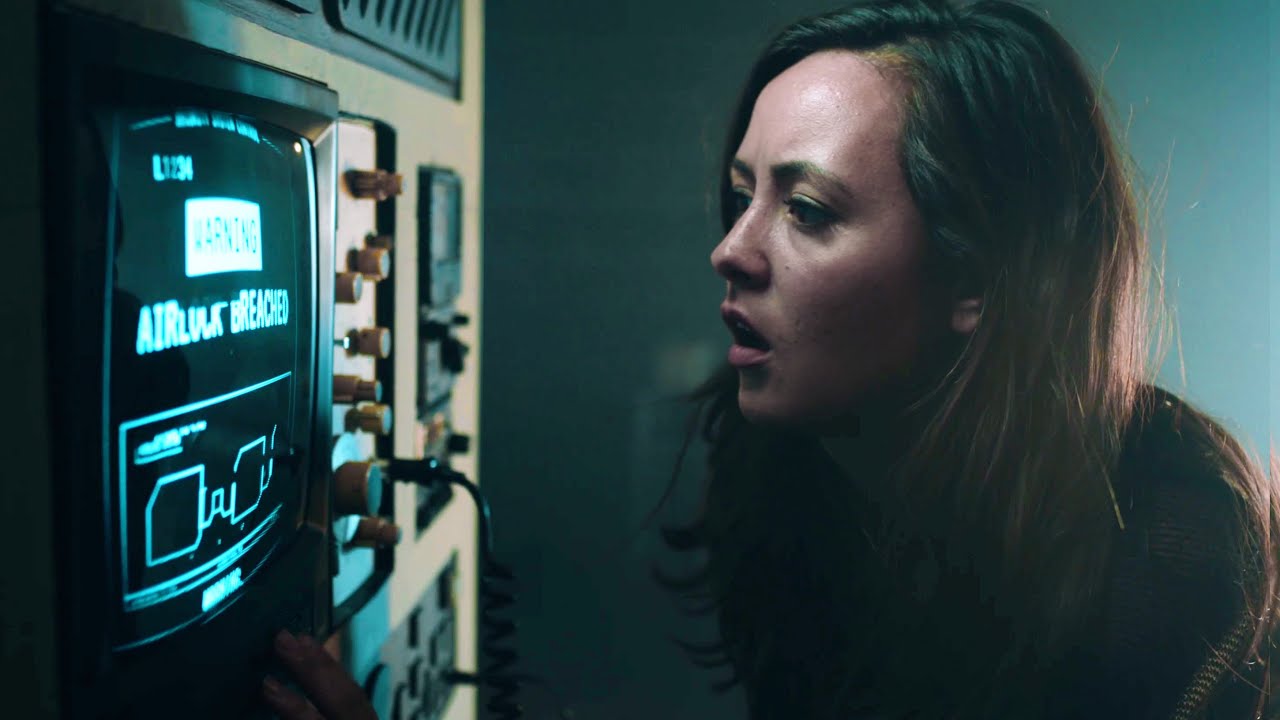This image captures a dramatic scene featuring a light-skinned woman with long, wavy brunette hair, parted on the left and flowing down past her shoulders. She appears surprised or concerned, her mouth slightly open, as she gazes intently to her right at a screen within a bank of complex instruments. The screen, reminiscent of 1980s television monitors, displays a black background with a bright teal message that reads 'WARNING: AIRLOCK BREACHED' in blue and white text, accompanied by various symbols and circuit-like imagery. Surrounding the screen are beige and brown buttons, switches, and twist knobs, along with yellow push-pull configurations and black plug-in wires, all contributing to the intricate appearance of the machinery. The background transitions from a bluish horror movie hue to a lighter teal in the upper right-hand corner, and the overall setting evokes the feel of an old factory or telephone switchboard. The woman, clad in a dark sweater or jacket, with eye makeup accentuating her features, stands slightly to the right of the image, her hand possibly near the machine, bringing together a sense of tension and urgency.